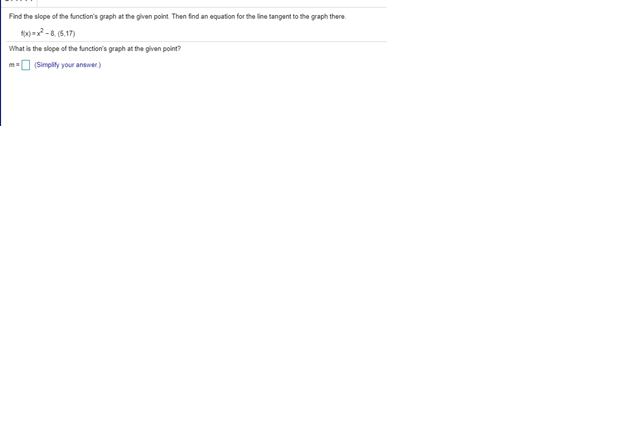The image is a screenshot from a computer, focusing on a small section of the screen. The background at the top of the image is solid white. A purplish-navy line appears on the left side. In black text, the instructions read: "Find the slope of the function's graph at the given point. Then find an equation for the line tangent to the graph there." Below this, the function is stated as \( f(x) = x^2 - 8 \), with a specific point noted in parentheses as (5, 17). A very faint gray line horizontally spans the width of the image, demarcating the next section.

In the subsequent part, the problem is reiterated, asking, "What is the slope of the function's graph at the given point?" Beneath this query, "m =" is followed by an empty white rectangle with a teal border. Next to the rectangle, a blue parenthetical note advises, "simplify your answer." The remaining portion of the image is completely white, emphasizing the focus on the mathematical problem.